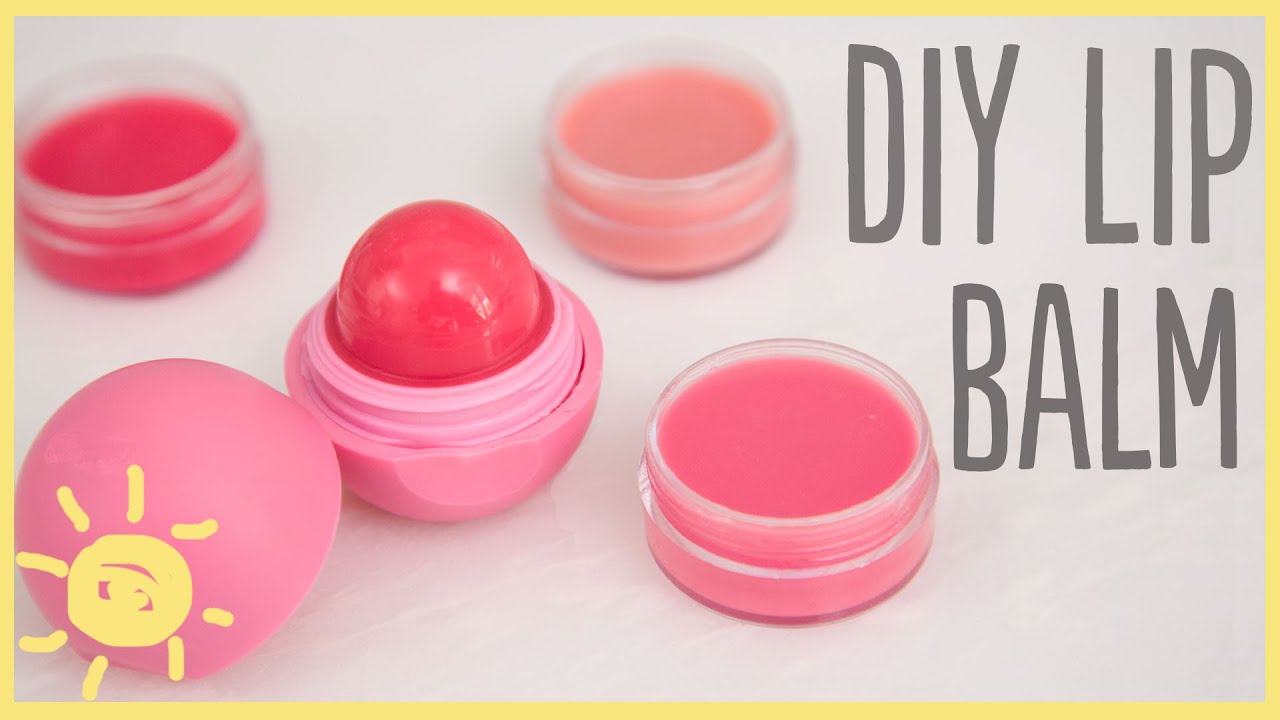The photograph features a DIY lip balm poster with a yellow border. The backdrop is a gradient from off-white to light gray. In the top right quadrant, the text “DIY lip balm” is prominently displayed in gray lettering. Below the text, three plastic containers of lip balm are showcased, each with oval-shaped, hard plastic cases in pink. The containers have flat bases and come in three shades: a deep red, a bright pink, and a peach. The bright pink lip balm is positioned in the center, flanked by the skin-colored peach to the top and the dark pink at the upper right. In the bottom left quadrant of the image, there is an upside-down, childlike drawing of a sun with a face, lending a whimsical touch to the composition.